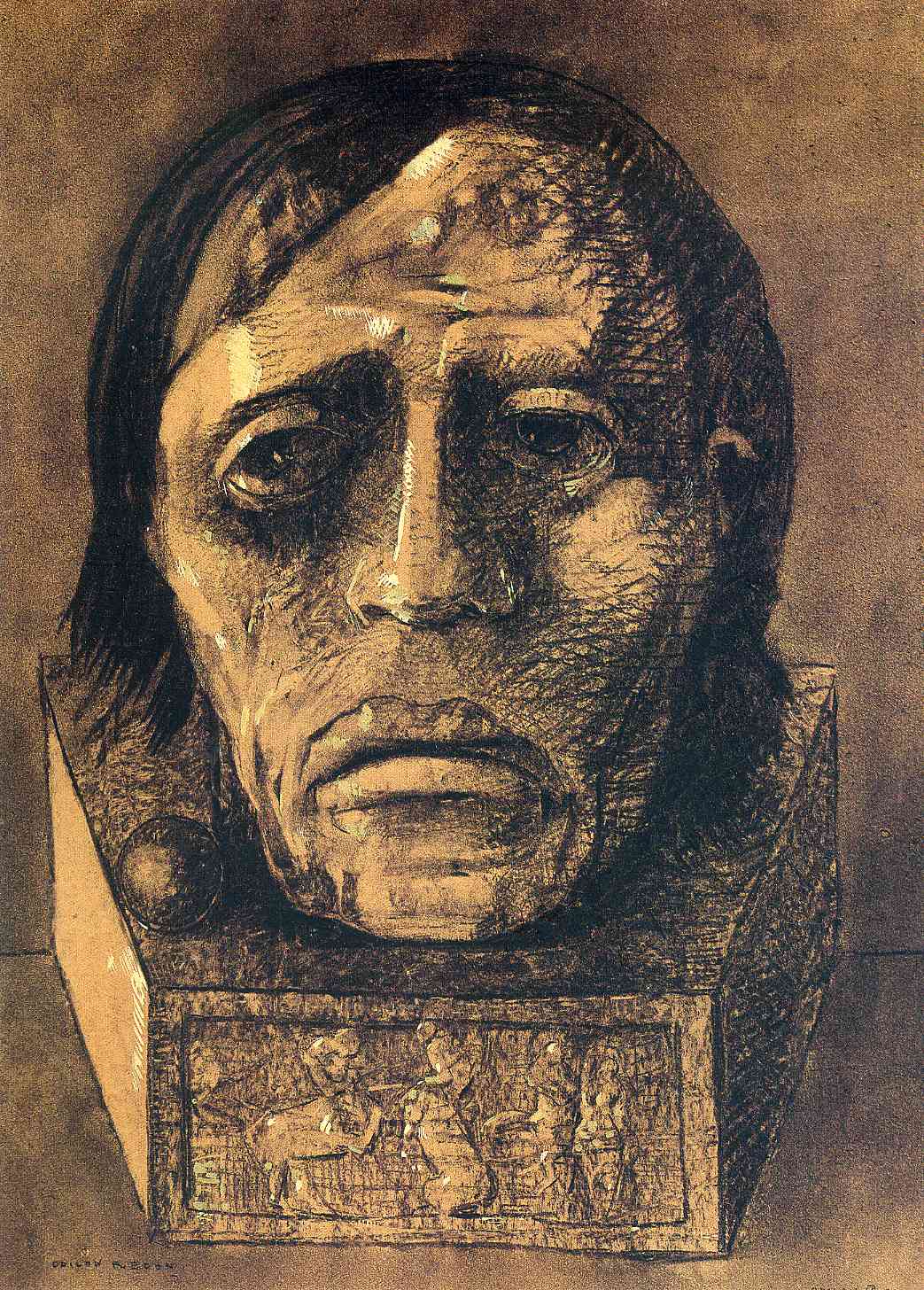The image depicts a detailed sculpture of a man's head with a somber expression, characterized by a downward-turning mouth and frowning eyes, almost giving the impression that he is crying. The man has dark black hair and is gazing off into the distance, although his face is oriented towards the viewer. The sculpture head is mounted on a uniquely shaped obelisk-like base. The base features intricate designs, including figures that resemble mythological creatures such as half-man, half-horse beings. Additionally, there is a metallic ball positioned to the right of the chin on the base. The entire image has a predominantly brown, beige, and black color palette, enhancing the ancient, almost Egyptian or Native Indian aesthetic of the artwork. The background remains simple, focusing attention entirely on the expressive head and its distinctive base.